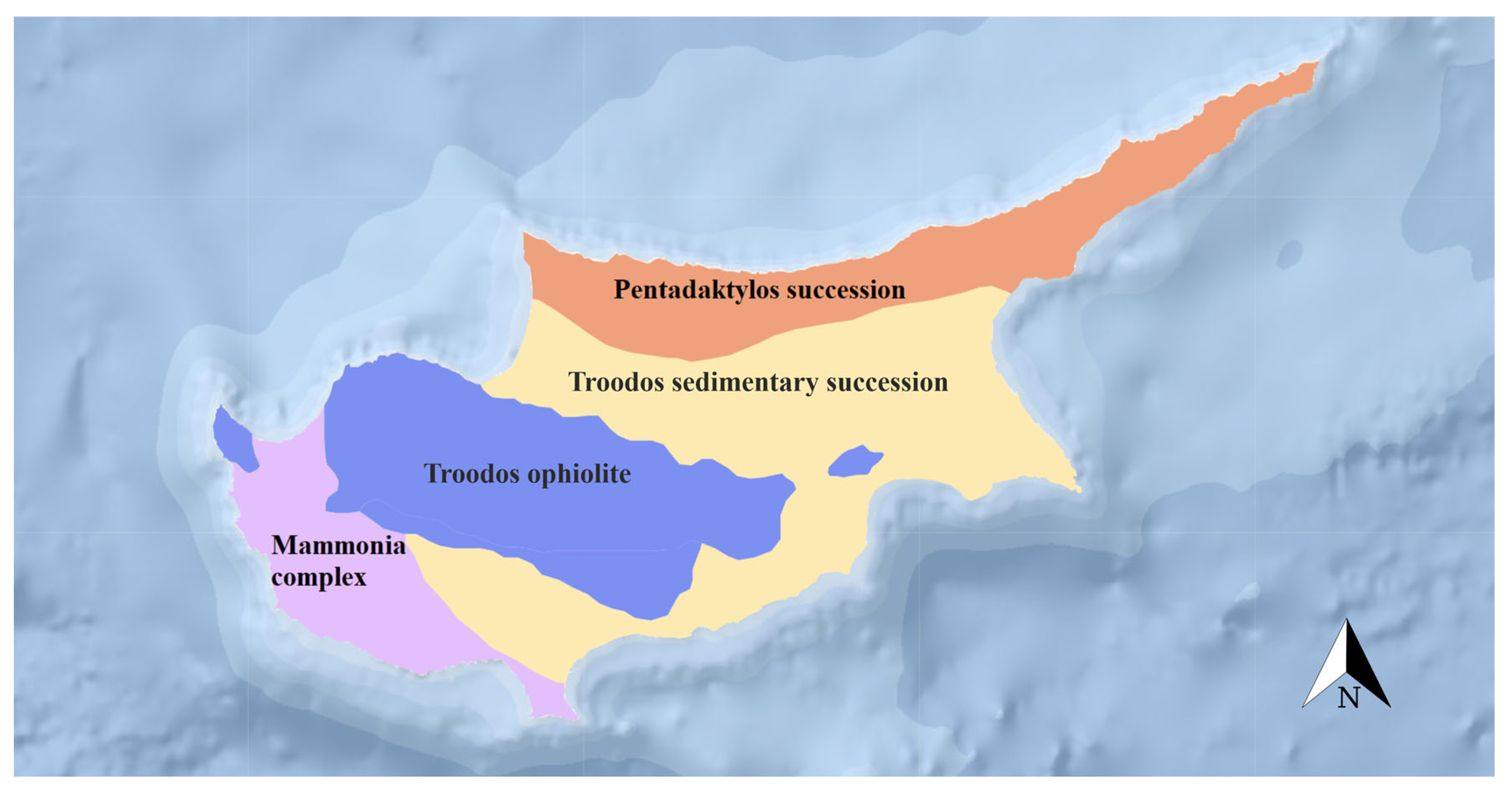This map features a north arrow in the bottom right corner, oriented upwards. The background predominantly consists of varying shades of blue, which portray a textured, almost mountainous terrain. At the center of the map, distinct colored strips from top down display different geological sections. 

First, a thin strip of peachy-orange labeled "Pentadactylus Succession" stretches nearly to the right-hand corner. Below this, a wider strip of yellow represents the "Trudos Sedimentary Succession," which dominates the map and encircles isolated patches of dark blue. This dark blue area signifies the "Trudos Aphelite." Finally, an expanse of pink labeled "Mammonia Complex" covers the bottom-most section, intersected by small strips of blue that appear sporadically within both the pink and yellow areas.